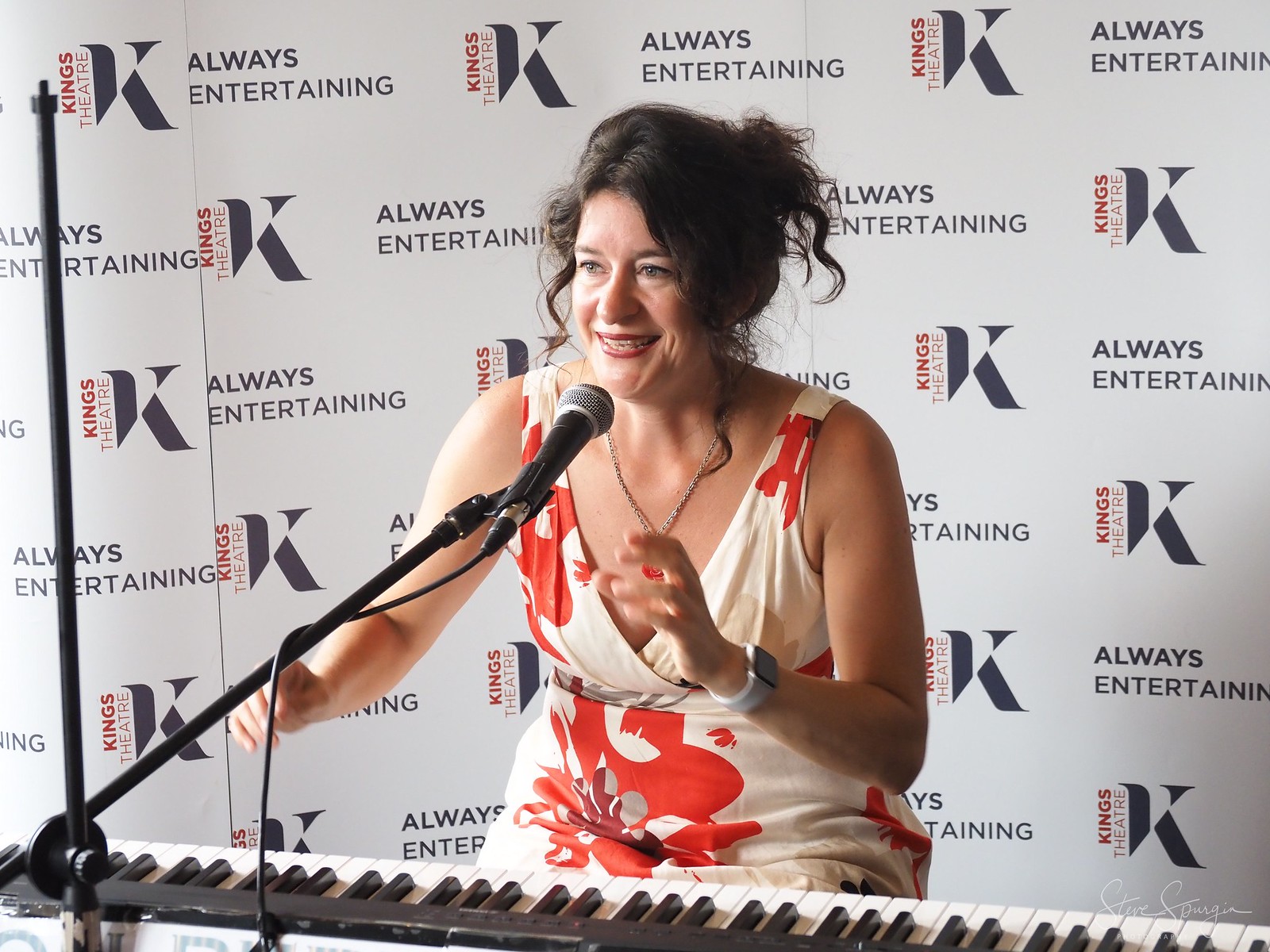In this detailed color photograph, a woman in her 40s or 50s is seated at a musical keyboard, smiling broadly with her teeth showing. She is facing slightly to the left, her dark hair pulled back into a loose, uneven bun. She wears a sleeveless white dress adorned with red floral patterns and a low-cut V-neck, complemented by a necklace with a red pendant. On her left wrist is a white-banded smartwatch or Fitbit. A silver and black microphone is positioned on a stand extending from the keyboard's left side, close to her mouth. Her left hand, slightly blurred, is gesturing near the microphone, while her right hand hovers above the keyboard's white and black keys, partially visible at the image's bottom edge. Behind her, a white wall features a repeating pattern of the phrases "Always Entertaining" and "King's Theatre," along with a prominent large 'K'. The words "King's Theatre" are written vertically beside each 'K' in red. The woman appears to be either performing or preparing to perform at King's Theatre, exuding a vibrant and joyful presence.